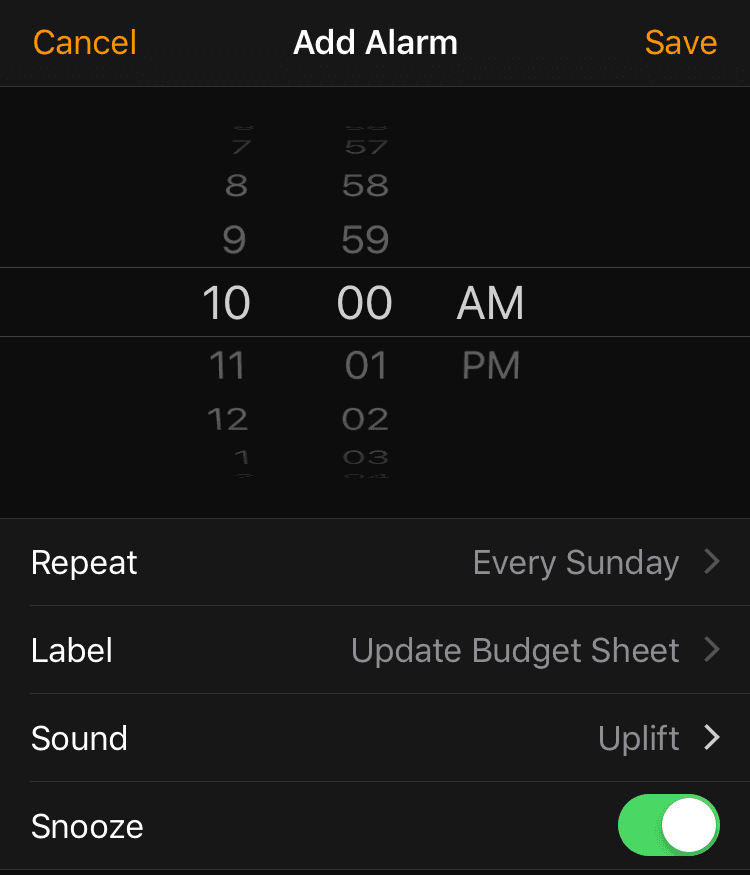The image depicts the interface for setting a new alarm on a mobile phone, displayed on a black background. At the very top in white text, it reads "Add Alarm." On the left top corner, there is an orange "Cancel" button, while the right top corner features an orange "Save" button.

Below this, the main focus is a rotary-style time selector, currently set to 10:00 AM. The selector allows you to individually adjust the hour, minute, and AM/PM settings by sliding them up and down. The digits 9, 8, 7, as well as 11, 12, and PM, are faintly visible around the current selection.

Further down is a set of additional options:
- **Repeat**: Set to "Every Sunday," which likely means the alarm will ring every Sunday.
- **Label**: Set to "Update the budget sheet," presumably indicating the purpose of this alarm.
- **Sound**: Set to "Uplift," suggesting this is the chosen alarm tone.

At the bottom, there is a toggle for the snooze function, currently turned on, represented by a green switch with a white circle.

Each option—Repeat, Label, and Sound—has a forward arrow beside it, indicating that these settings can be further configured.